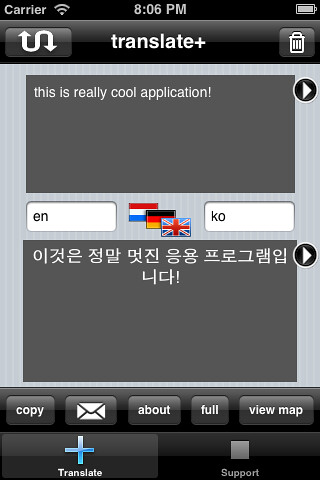The image is a screenshot of a phone display. At the top, there is a black banner displaying the carrier information on the left, a Wi-Fi signal icon, the time set to 8:06 PM in the center, and a fully-charged battery icon on the right. Below this top banner is another black and gray banner featuring an icon of arrows pointing up and down, labeled as "Translate Plus," and a trashcan icon to its right. The central part of the screen has a gray box with white text stating "This is a really cool application." Below this, there are two labels: "EN" on the left, with a flag next to it representing England, and "KO" on the right, with another flag, likely representing Korea along with Korean characters. At the bottom of the screen are several white buttons labeled "Copy," an envelope icon, "About," "Full," and "View Map." Beneath these is a blue button with a cross labeled "Translate" and another button labeled "Support" housed in a gray square.